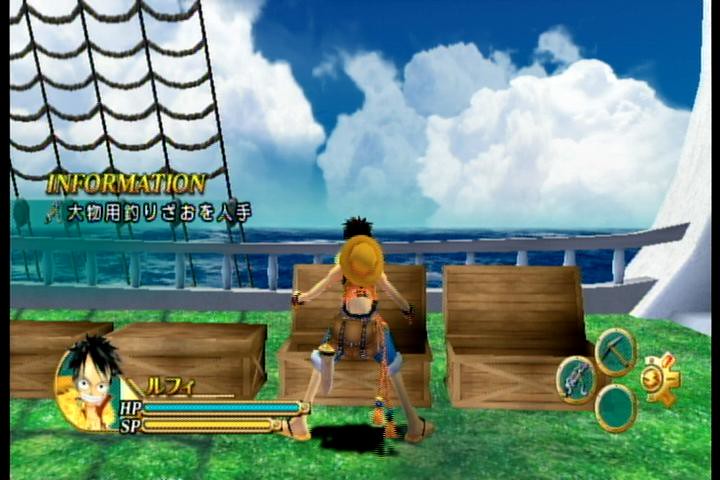The image is a detailed still from a fighter video game. It features a vibrant outdoor setting with a bright blue sky and large, puffy white clouds. The scene is set on a ship with astroturf-like grass covering its deck, bordered by netting and silver fencing. The left side of the image shows netting descending alongside the ship's side and masts, holding five pulleys.

At the center, a man with black hair, wearing blue shorts, flip flops, and a brown hat hanging on his shoulders, is opening a wooden crate. He has a black bag and two orange potion bottles hanging behind him. There are four wooden crates in the scene: two unopened crates to his left and an already-opened crate to his right. 

The bottom left corner of the screen displays the character's face with black hair, along with two progress bars: a blue HP bar and a yellow SP bar. To the right, four circles showcase various items, with one slot empty and another resembling a directional pad. Above the character information in the center-left, there is text labeled "information" with Chinese characters below it.